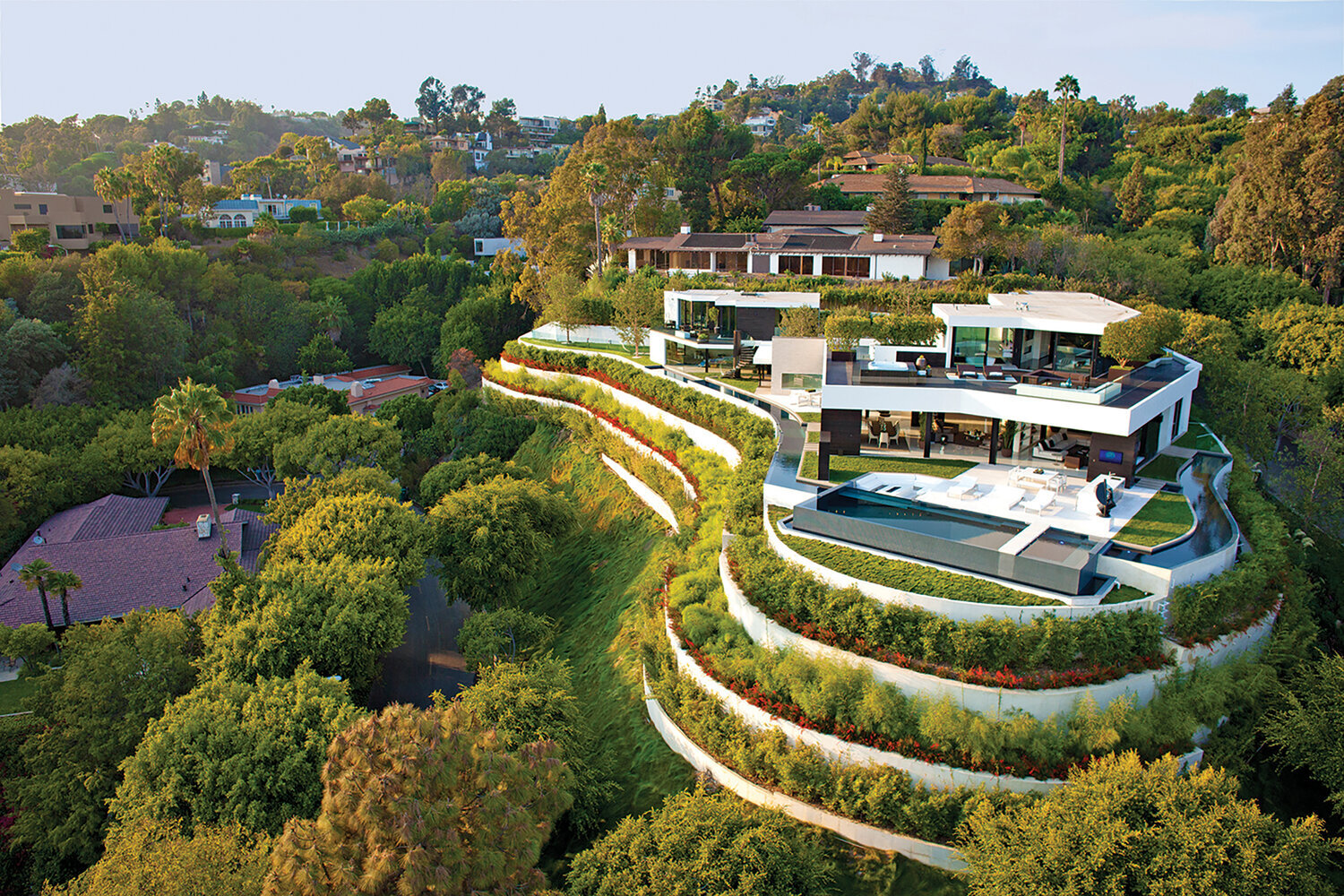The image depicts a luxurious contemporary mansion nestled on a hill, likely in California, surrounded by lush greenery and an array of trees, including evergreens, oaks, and palms. The elevated position of the house is supported by four tiers of retaining walls, adorned with vibrant red flowers and abundant greenery. The mansion features a strikingly open design, with large retractable walls that blur the line between indoors and outdoors. On the second level, there is a spacious deck adorned with trees, providing a serene vantage point. Additionally, there appears to be a guest house in the same architectural style, also buttressed by retaining walls. The property includes a shimmering pool at the top level, contributing to the sense of exclusivity and luxury. The sky overhead has a hazy white tint, accentuating the sunny and picturesque ambiance of the scene. Surrounding the mansion, other well-appointed houses are visible, cascading down the multi-leveled hills, each boasting expansive windows and sizeable backyards. The overall scene is one of opulence and architectural harmony, bathed in sunlight.